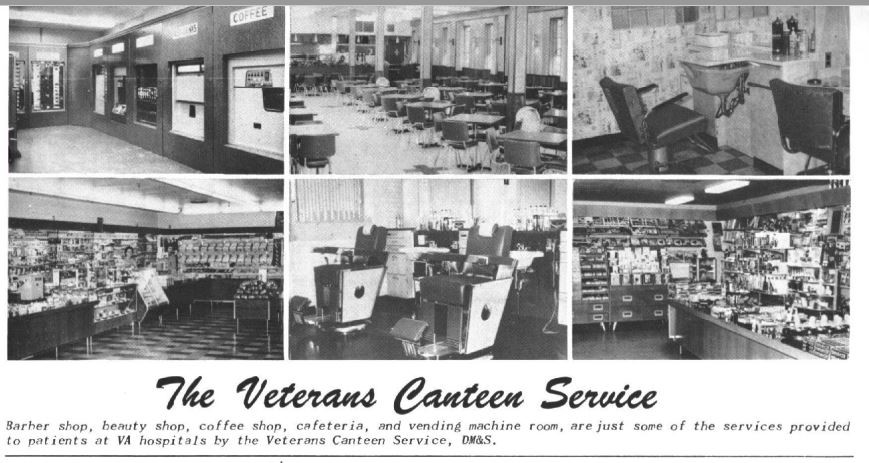This black and white horizontal image, approximately twice as long as it is tall, is divided into six equal-sized rectangular photographs, each depicting different areas inside the Veterans Canteen Service. It features scenes of a barbershop with a barber chair and sink, a beauty shop, a coffee shop with tables and chairs, a cafeteria, and a vending machine room. These photographs are separated by white borders. In the bottom third of the image, text reads, "The Veterans Canteen Service," followed by a list of provided amenities: barbershop, beauty shop, coffee shop, cafeteria, and vending machine room, which are available to patients at VA hospitals. The images mostly show empty rooms, adding to the clinical and orderly presentation typical of brochures or magazines aimed at informing patients or visitors about available facilities and services.